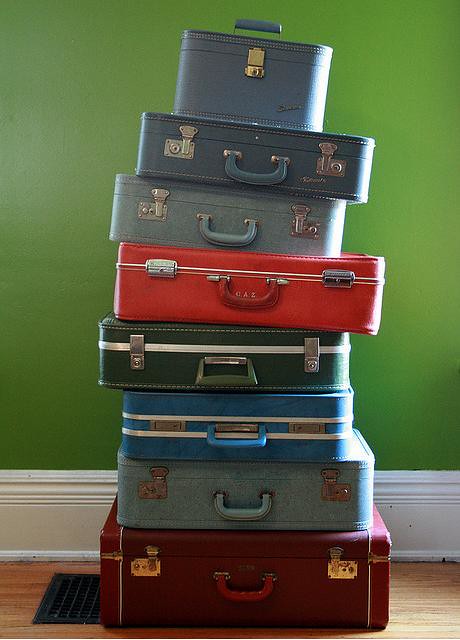This visually striking image, possibly an AI-generated creation, showcases a stack of eight vintage, old-school-style suitcases meticulously arranged on a polished wooden floor. The background features a vibrant apple green wall complemented by a wide, white, decorative baseboard, adding a nostalgic touch reminiscent of vintage homes. The suitcases, adorned with distinctive clasps and handles, are set on a small black mat and vary in color and detail, offering a rich palette including dark maroon, patterned dark grayish blue, blue and white, black with a white stripe, bright red with a white stripe, gray, and dark blue. Atop the stack sits a smaller, hatbox-like vanity case in dark teal. A black heating vent is visible on the floor to the left of the suitcase stack, further grounding the scene in a realistic domestic setting.